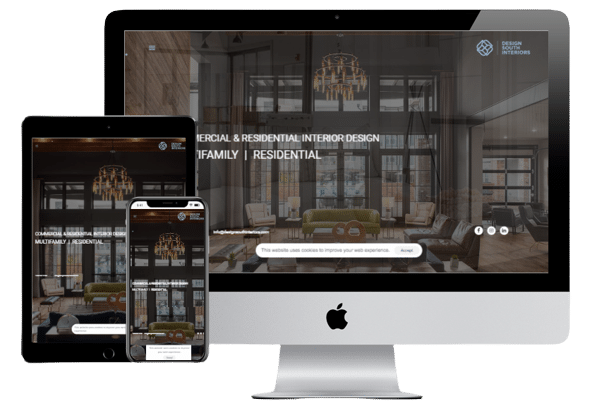The image features an Apple computer monitor with a sleek silver-gray base and a matching lower border. The sides and the top of the monitor are black, creating a distinctive frame around the screen. Displayed on the screen is an advertisement for "Commercial and Residential Interior Design." The visual within the ad showcases a sophisticated room with very tall windows and an elegant chandelier hanging from the ceiling. The room is furnished with a sofa, several chairs, and contains a certain type of box below a search bar, although its specific details are unclear. In addition, there are three indistinguishable icons to the right of the search bar. To the left of the computer monitor are a tablet and a smartphone, both displaying the same advertisement as the monitor. The tablet features a black border, whereas the smartphone has a gray border, complementing the color scheme of the monitor's base and bottom border.